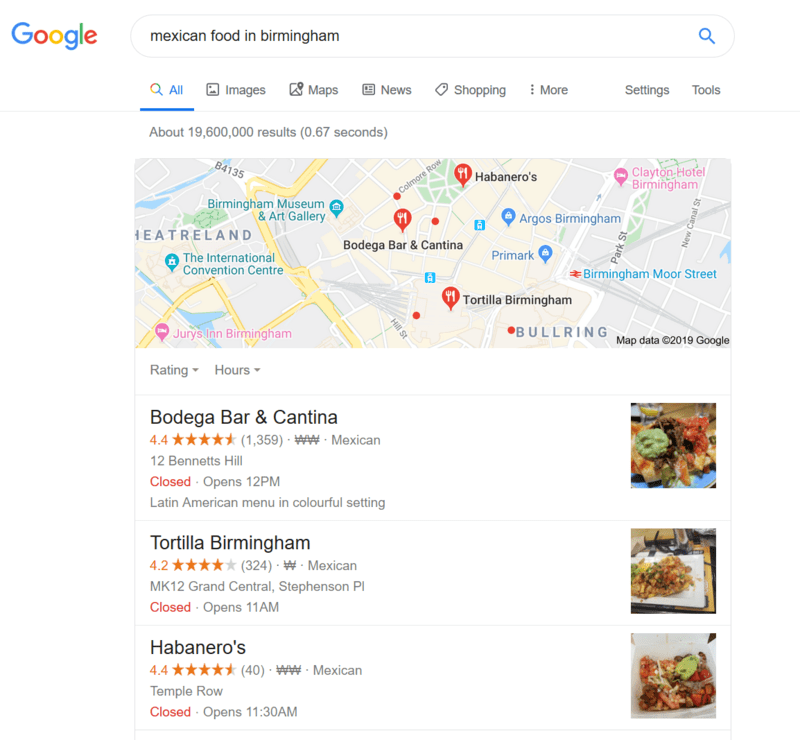The image depicts a search result page from a user querying "Mexican food in Birmingham." Horizontally aligned at the top of the page is the search bar containing the query, beneath which lies a map pinpointing the locations of various Mexican restaurants in Birmingham. The screen shows detailed information about three eateries, each currently closed, as indicated by a red "Closed" label.

The first result is Bodega Bar and Cantina, which boasts a 4.4-star rating based on 1,359 reviews. It's described as offering a Latin American menu in a colorful setting. The restaurant's address is listed, and it's noted that it will reopen at 12 p.m. The listing includes a thumbnail picture of the restaurant's food to the right.

The second result is Tortilla Birmingham, holding a 4.2-star rating from 324 reviews. It also identifies as a Mexican restaurant, located at MK-12, Grand Central. An image of some dishes presumably from the restaurant accompanies the listing.

The third spot highlighted is Habaneros, though specific details about its rating and reviews are cut off in the presented information. However, its location and the fact that it is also currently closed are visible. 

The map above shows pins indicating the precise locations of each restaurant, helping users visualize where they are situated within Birmingham.